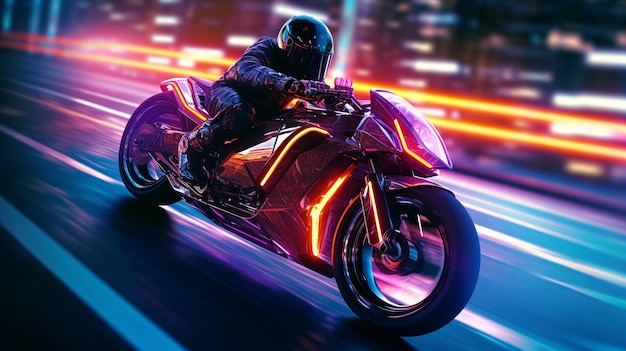The image depicts a possibly computer-generated scene of a person riding a sleek, futuristic motorcycle at high speed through a city street. The rider, dressed in a black helmet and black riding suit, is hunched down towards the handlebars, emphasizing the velocity of movement. The motorcycle is predominantly black, featuring glowing purple and fiery yellow-orange elements that add to its high-tech appearance. The background showcases blurred city buildings and streaks of motion, with the road appearing as a blur of white and yellow lines, reinforcing the impression of rapid travel. The overall lighting and vivid colors, along with the sense of motion, suggest that this image might be a digital creation rather than a real photograph.